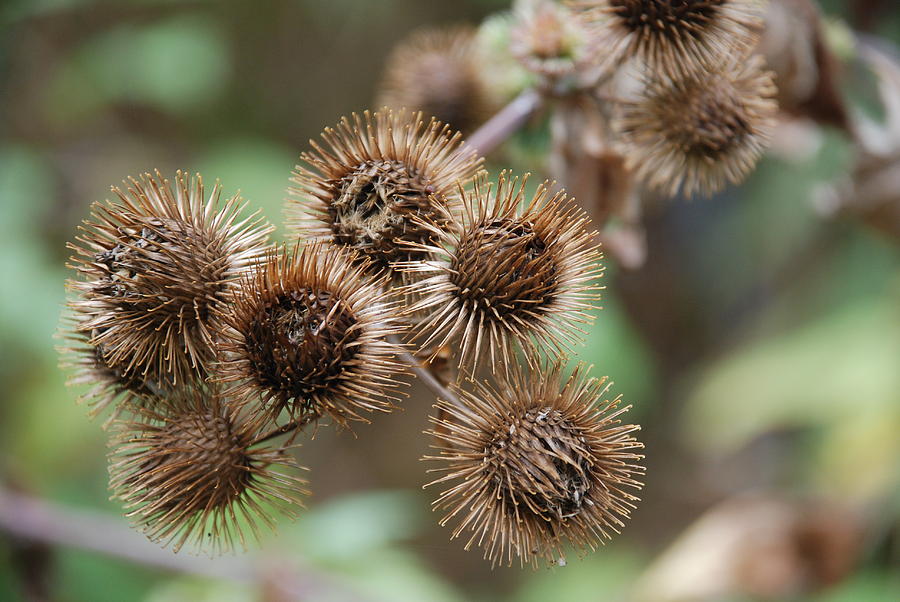This is a close-up photograph of a withered plant, often referred to as a 'stinging meadow' flower, characterized by its round, spiky brown pods resembling tiny, dried porcupine spheres. Each spiked bud extends from a main branch with multiple tiny offshoots, giving an overall appearance similar to a coronavirus model. The spikes are about an inch long, arranged in all directions, and some buds appear to be opening despite their dead or dying state. The background of the image is blurred, filled with varying shades of green and hints of brown and yellow, suggesting a mix of alive and decaying foliage, possibly indicating an autumn setting. The cloudy ambiance contributes to the subdued, muted tone of the scene, with no direct sunlight adding to the somber mood of the photograph.